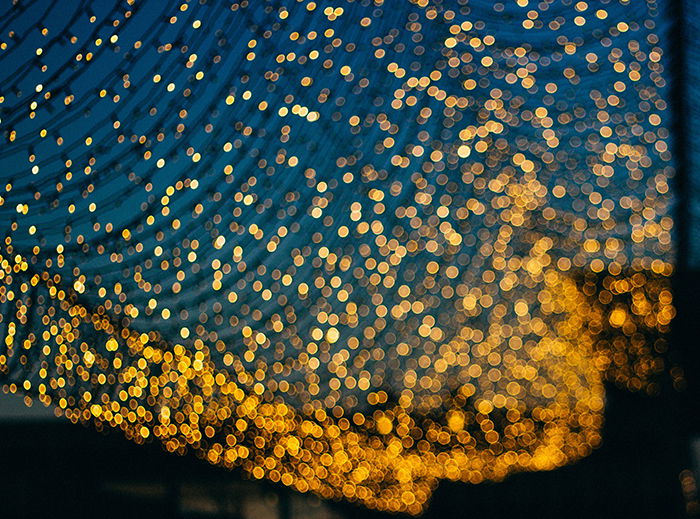The image depicts an abstract close-up view of numerous small, gold and bright yellow lights scattered against a smooth, satin-like blue background. The lights are mounted on a black, curved, metallic structure that appears to taper off at the bottom right corner. The gold and yellow lights are more concentrated and blur together forming a dense, almost indistinguishable mass in the bottom right corner, where the background turns completely black. Towards the upper left corner, the lights are more sparse and individually distinguishable, revealing more of the blue background. The lights give an impression of delicate fiber-optic points, especially clear on the left and bottom edges where they transition into a glowing blur on the right.